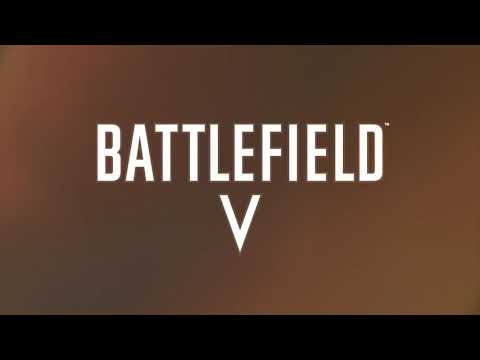The image is an edited or animated screenshot of the Battlefield V logo. The background features a blotchy pattern with varying shades of brown, transitioning from a lighter brown on the edges to a darker brown in the center, giving it a gradient effect. At the top and bottom of the image, there are black bars running horizontally from one side to the other. Centered in the image is bold, large, white block text in all capital letters reading "BATTLEFIELD," with the letter "V" directly beneath it, signifying the Roman numeral for 5. The "V" is aligned with the letters "L," "E," and "F" above it. Additionally, there is a small trademark symbol located above the "D" in "BATTLEFIELD."